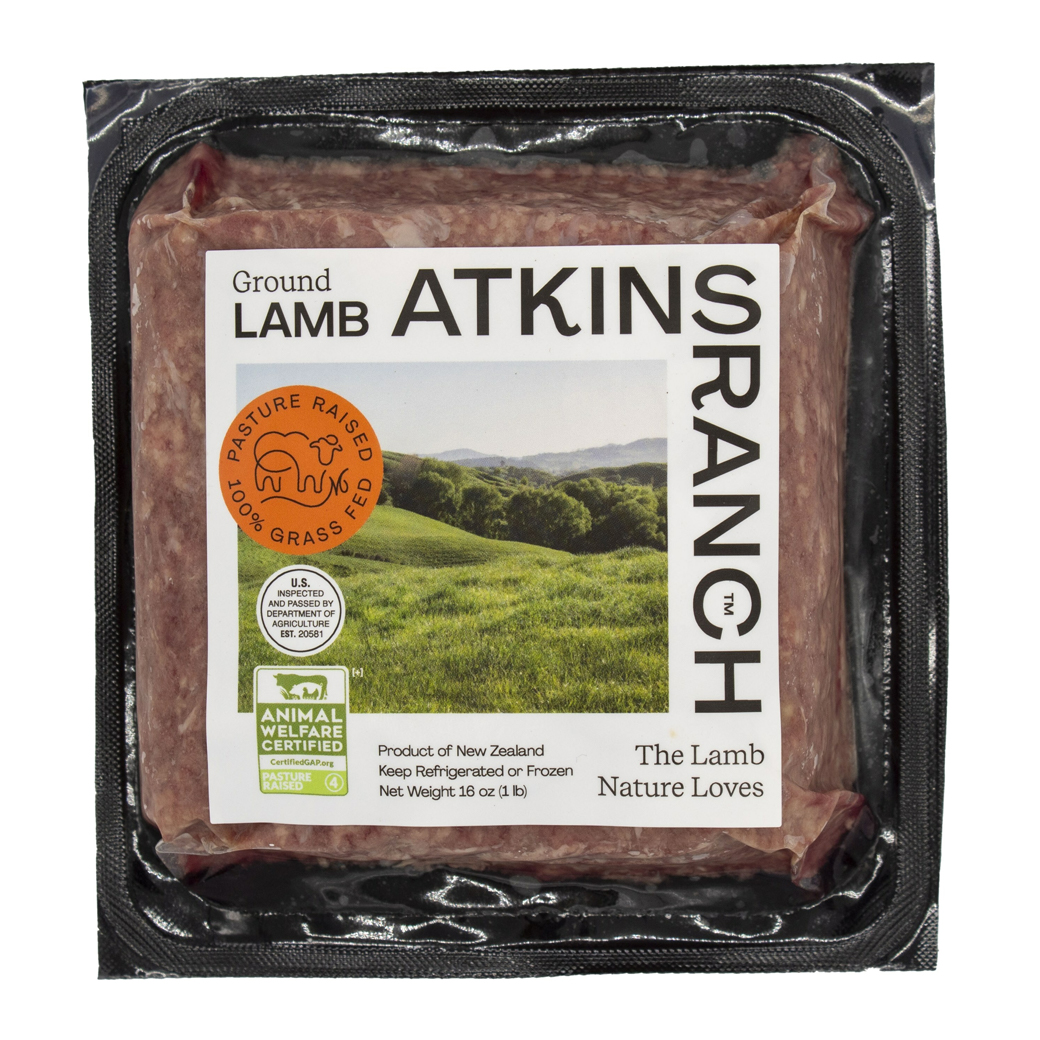This is a detailed photograph of a package of ground lamb from Atkins Ranch, presented on a pure white background. The package features a black square base, with a flush, dotted black line rounded at the corners. The ground lamb inside is shaped in a square and has a pinkish-brown color with white flecks, all encased beneath a glossy plastic covering. 

On top of the package is a prominent white square label. At the center left of the label is an image depicting a lush, green rolling hilly landscape with a forest and a distant line of mountains. The black text across the label reads "Ground Lamb" at the top, followed by "Atkins Ranch" and "The Lamb Nature Loves" to the right, rotated 90 degrees. Further details include "Product of New Zealand", "Keep Refrigerated or Frozen", and "Net Weight 16 oz." (1 pound). 

The label also features three badges on its left side. The top badge is an orange circle stating "Pasture Raised 100% Grass-Fed" with a black illustration of a lamb. The middle badge is a white circle with black text saying "US Inspected and Passed by Department of Agriculture EST 2581." The bottom badge is a white and green design showing a green silhouette of a cow and a chicken, with "Animal Welfare Certified" in white text, and "Certified GAP.org" in green text beneath, finished with "Pasture Raised."